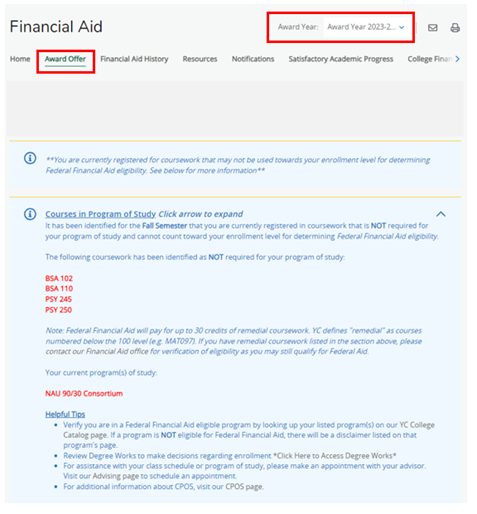The image showcases an interface for a financial aid portal, with various navigational and informational elements presented on a structured layout. 

**Top Section:**
- **Header**: At the top left, prominently displayed text reads "Financial Aid."
- **Contextual Bar**: Adjacent to this, aligned to the right, there is a red-outlined rectangle containing the text "Award Year: 2023-2," followed by a dropdown blue arrow. This same section also includes icons for email and printing, indicating functional actions.
  
**Navigation Menu:**
- **Options**: Below the header, there's a horizontal navigation menu featuring several clickable items:
  - Home
  - Award Offer (Highlighted in green with a red box around it)
  - Financial Aid History
  - Resources
  - Notifications
  - Satisfactory Academic Progress
  - College
  - FI (followed by a right-facing arrow)
  
**Notification Section:**
- **Alert Box**: Moving down into the blue-background area, an informative icon precedes a critical message in a yellow-outlined box. The message reads: "You're currently registered for coursework that may not be used towards your enrollment level for determining federal financial aid eligibility. See below for more information."

**Course Information:**
- **Expandable List**: This section also includes elements labeled "Courses and Program of Study," with an arrow indicating expandability. Listed courses include details of the "NAU 90-30 Consortium," with specific course numbers highlighted in red for emphasis.

**Additional Resources:**
- **Footer Information**: Finally, the section ends with a note on "Helpful Tips" displayed in blue, providing users with quick assistance in navigating or understanding the process. 

This detailed layout emphasizes ease of access and clarity for users managing their financial aid details.